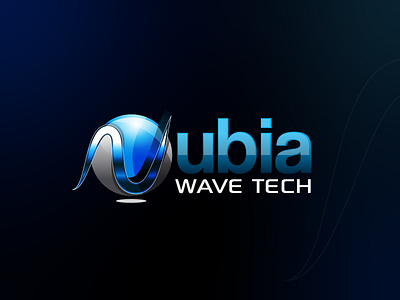The image features a logo set against a black background. The logo comprises a stylized letter "U" over a blue and silver globe, with a small white square at the bottom of the globe that could be part of the design or a shadow. To the right of this globe, the text "UBIA" is displayed in lowercase letters, with a light blue gradient at the top transitioning to a grayish blue at the bottom. Below "UBIA," the phrase "WAVESPACE TECH" appears in all capital, white letters. The "U" in the logo looks like it is integrated into the globe design and may cast a subtle shadow. The fonts are both sans serif, with "WAVESPACE TECH" being slightly smaller. The overall composition hints at a technology-related company.